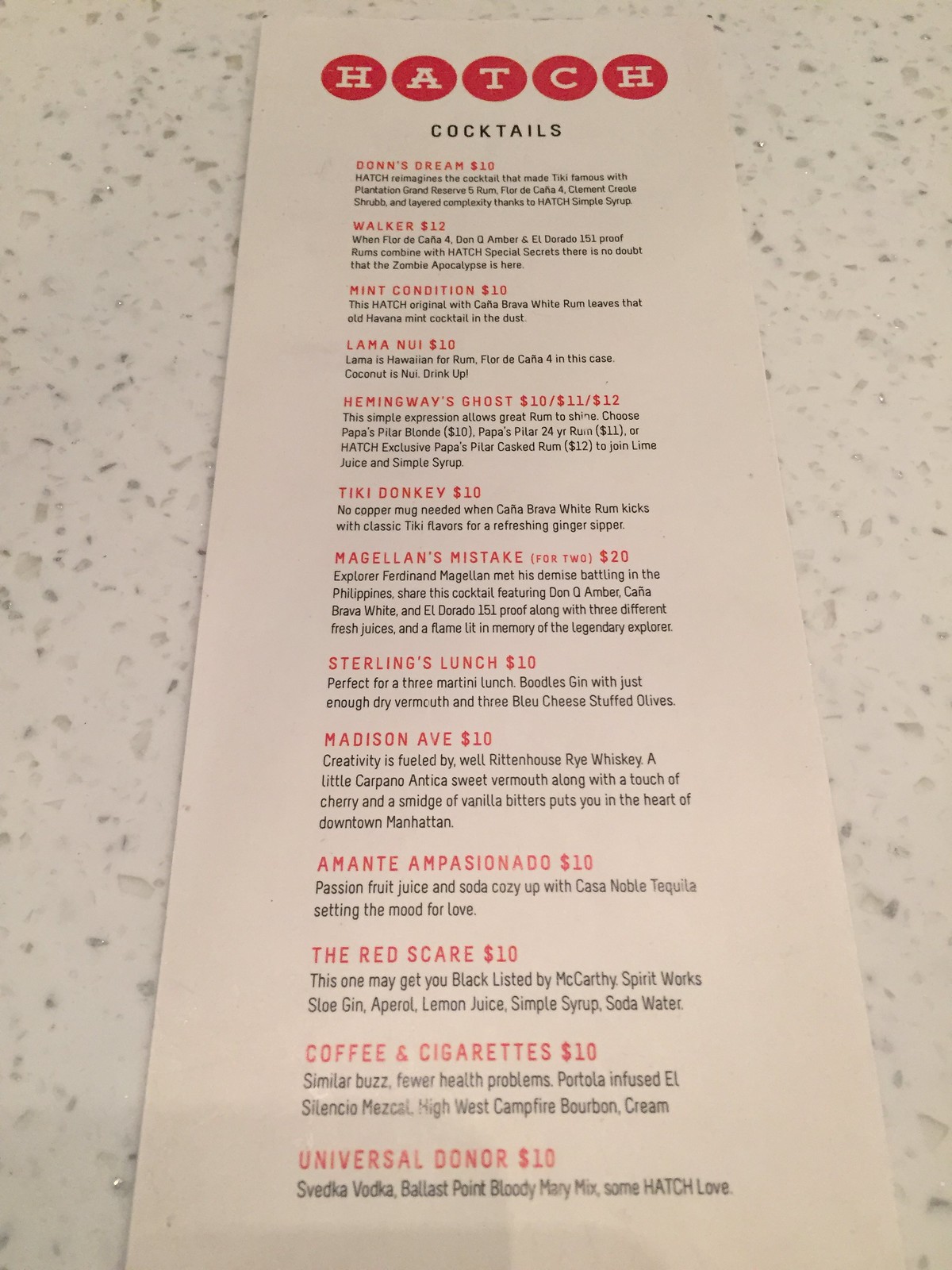The image captures a menu laid flat on a countertop, viewed from a low angle as though the photo was taken from the bottom edge of the menu. The countertop appears to be made of white quartz or granite, adding a clean and sophisticated background to the image. The menu itself features a white background with the letters "HATCH" prominently displayed at the top, each letter enclosed in a red circle with white lettering. Below "HATCH," the word "COCKTAILS" is written, followed by a list of mixed drinks.

The menu includes a variety of creatively named cocktails with brief descriptions and prices. At the top of the list is "Dawn's Dream" priced at $10, described as HATCH's reimagined version of the classic Tiki cocktail. Next is "Walker" for $12. The "Mint Condition" is another $10 option, branded as the HATCH Original with Caja Brava White Rum, promising to leave the traditional ETD Havana Mint Cocktail behind. "Llama Nui" also comes in at $10, followed by "Hemingway's Ghost," a rum-based drink noted for its simple expression that lets great rum shine. Other cocktails include "Madison Ave," "The Red Scare," and "Coffee and Cigarettes," all priced at $10 each.

The drinks are described succinctly, implying a mix of both classic and innovative flavors, presented in a stylish and modern menu design. The image captures the essence of an upscale cocktail bar setting.